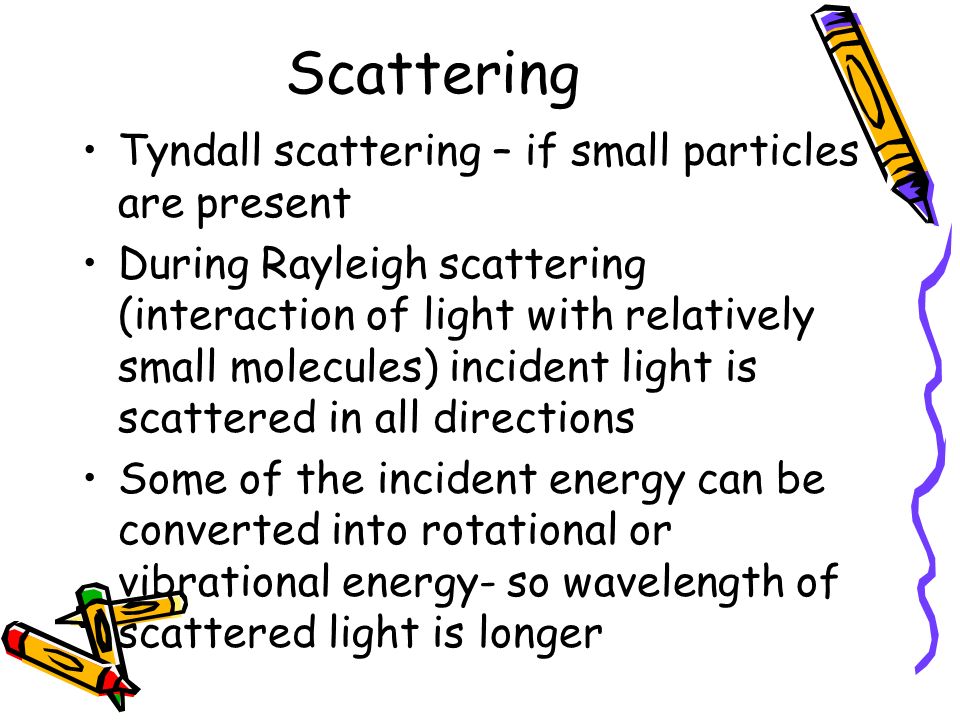The image features a predominantly white background with black text describing the properties of light scattering. At the top, in bold, larger font, is the title "Scattering". Below this, a series of bullet points delve into different types of scattering: 

1. "Tyndall scattering" explains how light is scattered when small particles are present.
2. "Rayleigh scattering" is detailed as the interaction of light with relatively small molecules, where the incident light is scattered in all directions.
3. Another point mentions that some of the incident energy can be converted into rotational or vibrational energy, resulting in a longer wavelength of scattered light.

Visually, the image includes a few colorful elements: in the bottom-left corner, there are three crayons—red, green, and yellow—all featuring yellow wrappers with black ovals. On the right side, a purple crayon with a gold wrapper is depicted, drawing a wavy line from the bottom to the top of the page. This purple line intersects and winds through the text, adding a whimsical touch to the informative graphic.